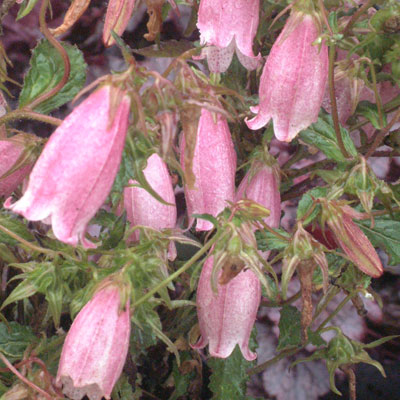This photograph captures a close-up view of a flowering vine adorned with an abundant display of bellflowers, also known as campanulas. Each flower, in shades ranging from light to medium pink with subtle white highlights near the tops, hangs downward, resembling delicate bells. The bellflowers are mostly in full bloom, though some remain tightly closed, hinting at the plant's continuous blossoming cycle. The foliage, featuring green leaves and stems with a slight red tint, interweaves with the flowers, adding a muted green backdrop to the vivid flora. Scattered amongst the visible 8 to 15 prominent flowers are additional buds and blooms, indicating the lushness of the entire plant. Although the supporting structure such as a trellis or possibly the side of a house is implied, it is not captured within the frame, ensuring the viewer's focus remains solely on the intricate beauty of the flowers and greenery.